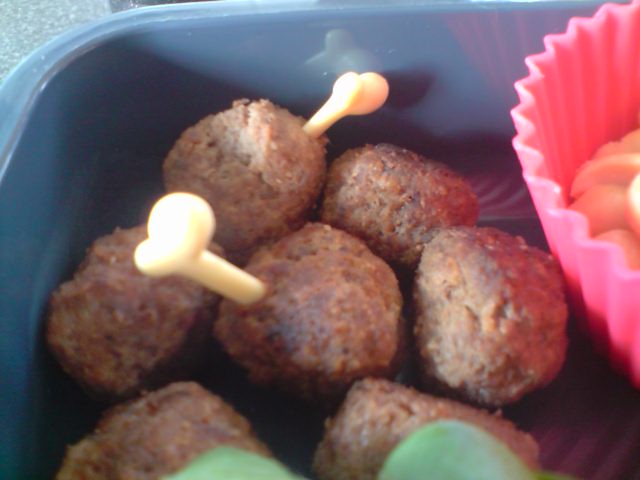In this close-up image, a tall blue or green plastic tray is seen holding seven spherical, charred, and cooked meatball-like items, each roughly three inches in diameter. Arranged in a circular pattern with one in the center, these balls appear to be bean-based or falafel-like rather than cheese or meat, and two of them have long, white plastic bones or toothpick-like utensils stuck in the middle, presumably for easy handling. To the right of the tray, there is a pink cupcake holder containing what looks like a minimal amount of white frosting or possibly peanuts. Additionally, the bottom center of the image reveals the tips of two green leaves.